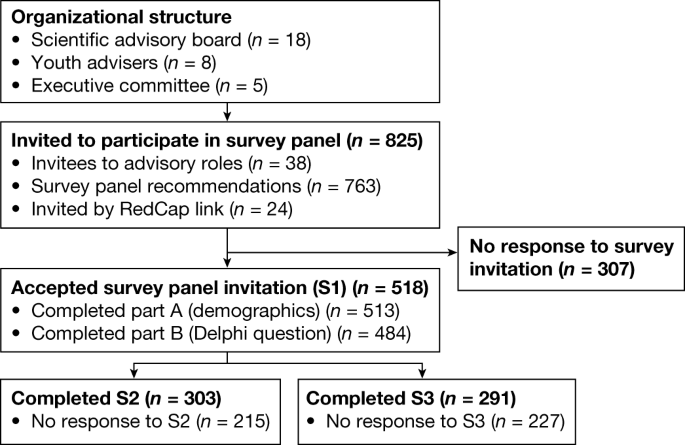This black and white flowchart outlines the organizational structure and survey process of a particular study. At the top, the main box is labeled "Organizational Structure," featuring three bullet points: Scientific Advisory Board (N = 18), Youth Advisors (N = 8), and Executive Committee (N = 5). An arrow points down to the next box labeled "Invited to Participate in Survey Panel" (N = 825), which lists three bullet points: Invitees to Advisory Roles (N = 38), Survey Panel Recommendations (N = 763), and Invited by Red Cap Link (N = 24). An arrow from this box leads to another labeled "Accepted Survey Panel Invitation S1" (N = 518), with sub-points indicating those that completed Part A: Demographics (N = 513) and completed Part B: Delphi Question (N = 484). A side arrow from the "Accepted Survey Panel Invitation S1" box notes "No Response to Survey Invitation" (N = 307). Below, the chart splits into two boxes: the left box shows "Completed S2" (N = 303) with "No Response to S2" (N = 215) noted underneath, while the right box indicates "Completed S3" (N = 291) with "No Response to S3" (N = 227). The flowchart effectively details the study's participant structure and survey response outcomes.